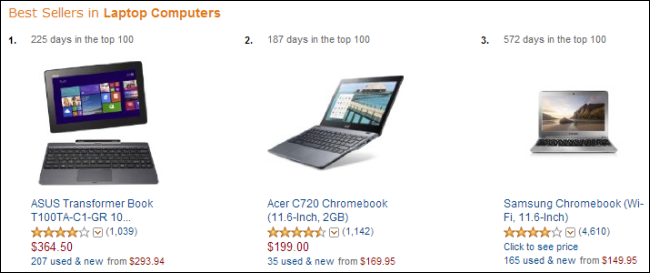The image showcases a selection of the three best-selling laptop computers, likely from an ecommerce platform. A black-outlined rectangle highlights this section, with a gold-orange header reading "Bestsellers" followed by a bolded "Laptop Computers" in the same hue. Three products are listed beneath this.

1. The first product has maintained a position in the top 100 for 225 days. It features an image of a laptop with a detachable screen, resembling a tablet. The product is the ASUS Transformer Book T100TA-C1-GR. Partial details indicate it has a 4 out of 5-star rating from 1,039 reviews, denoted by a gold drop-down arrow. The price is $364.50 in red. Below this, in blue, it mentions "207 used & new" from $293.94.

2. The second best-seller has been in the top 100 for 187 days. It displays a conventional laptop with a grey chassis and a screen showing a tropical hut over water. The model is the Acer C720 Chromebook, 11.6-inch with 2GB of RAM. It boasts a 4.5-star rating from 1,142 reviewers, shown with a gold arrow. The price is marked as $199 in red, with "35 used & new" from $169.95 in blue.

3. The third laptop, reigning in the top 100 for 572 days, exhibits a light silver chassis with a beach sunset scene on the screen and black keyboard keys. It's labeled as the Samsung Chromebook, Wi-Fi, 11.6-inch. It has earned 4 out of 5 stars from a substantial 4,610 reviews. The price is listed as "Click to see price", with "165 used & new" from $149.95 in red.

This detailed listing provides comprehensive information on each of the top three best-selling laptops, reflecting customer reviews, duration in the top charts, prices, and availability of used and new units.